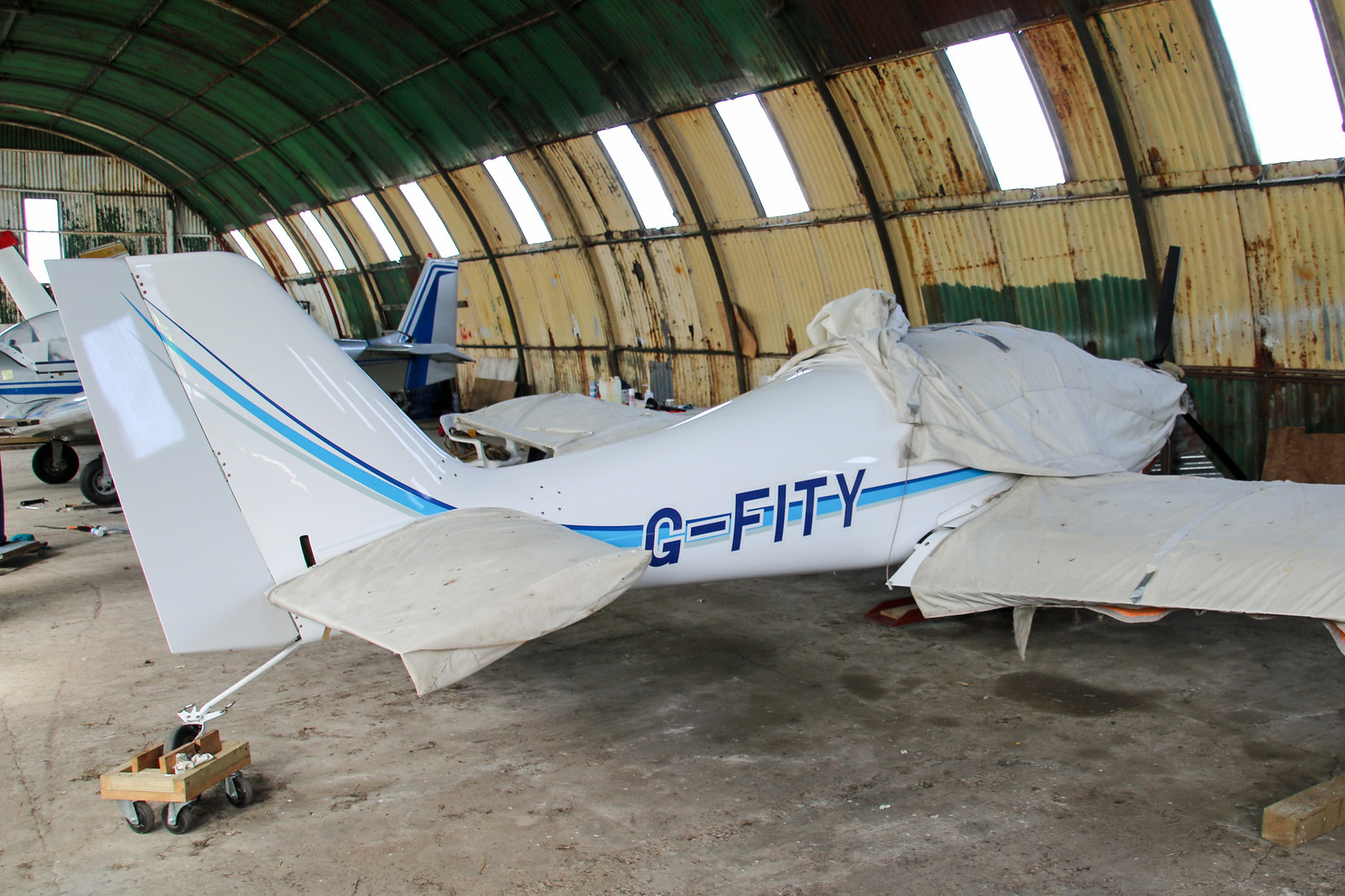This full-color photograph captures the interior of a very old, rusty airport hangar with curved walls and a green roof. The hangar walls are predominantly yellow and adorned with large, brightly lit windows, suggesting daylight outside. Dominating the scene is a small, single-engine aircraft, possibly a Cessna, with the registration G-FITY painted in blue on its sleek white body. The aircraft's wings and front are partially covered with tarps, obscuring much of its structure. A distinct blue and silver striping pattern adds a touch of color to its otherwise standard appearance. Behind the tail of this plane is a small, wheeled cart, potentially used to maneuver the aircraft within the hangar. On the left side of the image, one can see parts of another plane, hinting at the busy yet dilapidated state of the space.